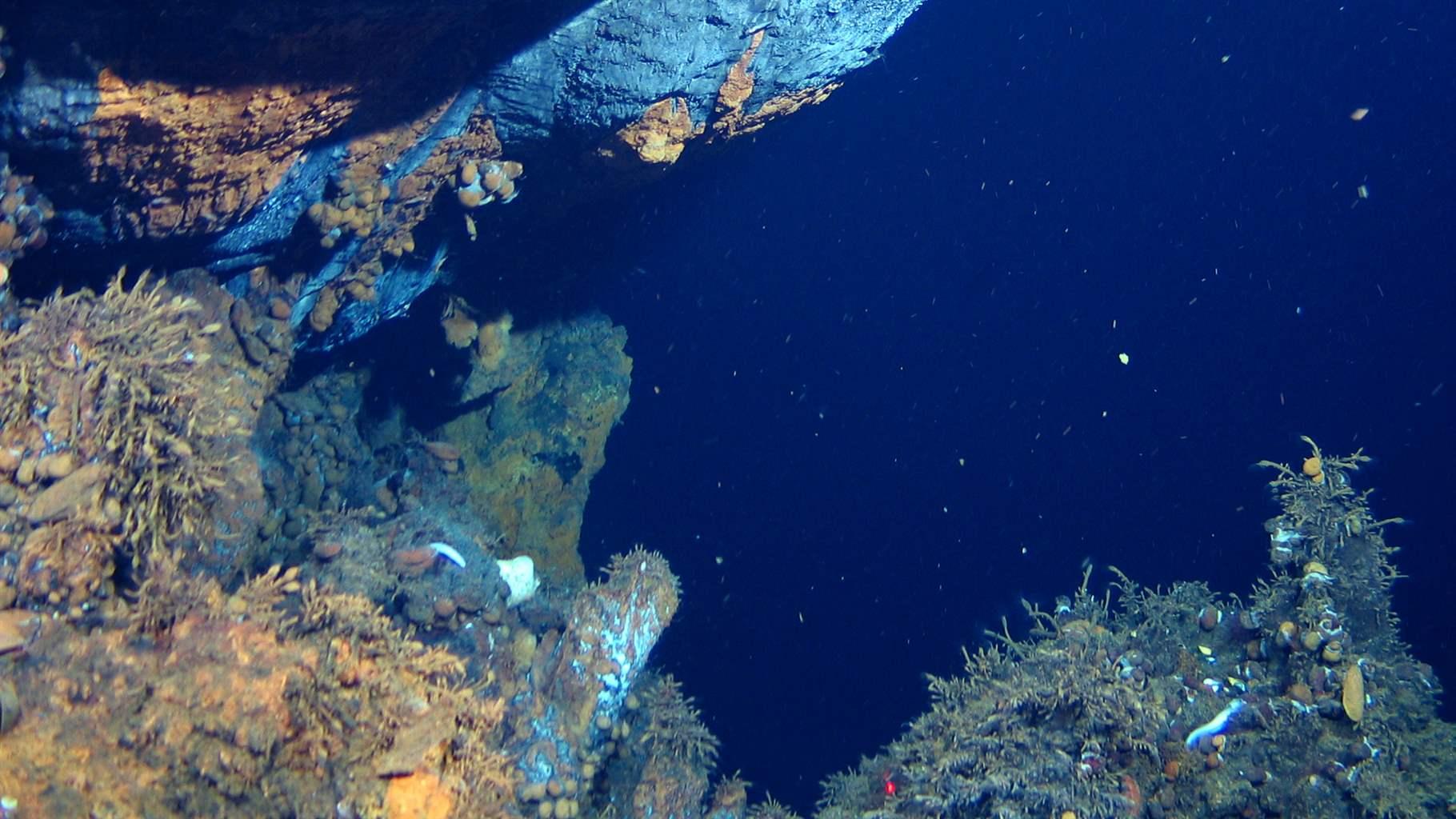The photograph depicts an underwater scene with a vibrant blend of colors and marine elements. The background is an expansive blue, suggesting deep ocean waters, accentuated with white, yellow, and green specks scattered throughout, likely particles suspended in the water. The image is illuminated, revealing a rock formation that dominates the upper left portion of the frame. This rock has a mix of colors, including shades of light blue and yellow on top, transitioning into orangey, green, and brown tones as it descends. The coral, appearing branch-like and plentiful, sprawls across the left side of the image, showing hues of orange and subtle flecks of red, blue, and yellow. On the right, the coral presence diminishes, limited to the bottom right corner, with the remainder of this side displaying a dark blue void dotted with small flecks. The overall scene captures a detailed coral reef, set against a geologically diverse underwater landscape, bathed in light, yet void of visible aquatic life.